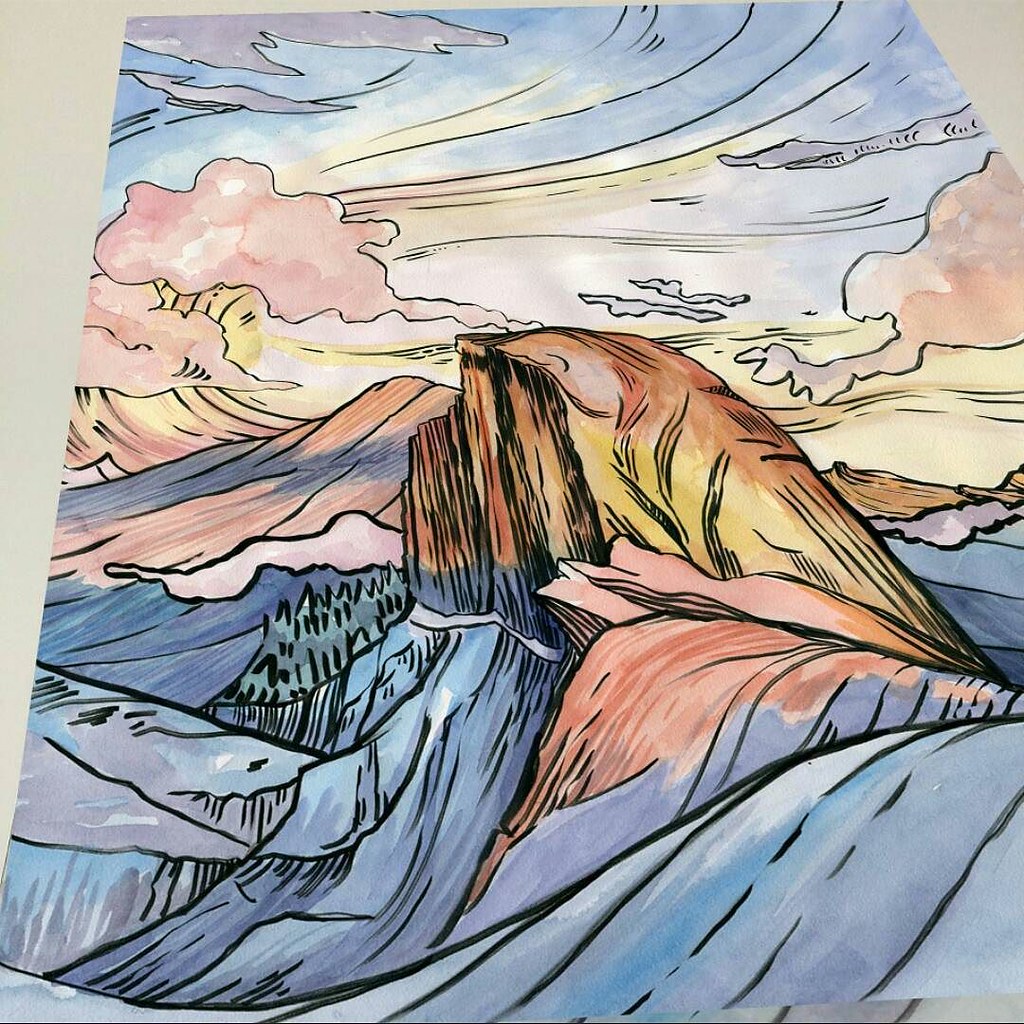A mesmerizing illustration-style artwork that captivates with its intricate details and vibrant color palette. At the center, a large rock outcropping stands prominently, adorned with hues of rust, blue, and yellow. This geological formation is surrounded by an array of majestic mountains painted in shades of rust, pale pink, deep and light blue, and subtle purple tones, all intricately outlined with fine black lines. Above this breathtaking landscape stretches a sky awash in a symphony of colors—light blue, yellow, purple-gray, pink, and orange gradients intermingling seamlessly. Wispy, pink-tinted clouds drift through the sky, adding a dreamlike quality to the scene. Encircling the rock outcropping, patches of green trees provide a touch of verdant life to the vibrant, almost surreal tableau.